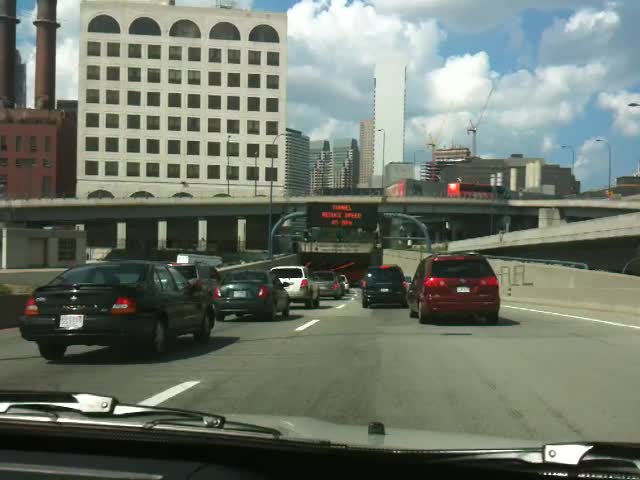The photo captures the view from inside a car, looking through the front windshield on a bright, sunny day. The vehicle is on a two-lane road marked by white dotted lines separating the lanes and is approaching a tunnel that runs under an overpass, leading into a large city. The road is busy with traffic in both lanes; visible ahead are a red minivan directly in front, followed by a black SUV and several other cars. In this car, windshield wipers and the vehicle's hood are in view. Above the tunnel entrance hangs a black marquee sign displaying an illegible message in orange text. Towering skyscrapers of the cityscape can be seen in the distance, set against a vibrant blue sky filled with fluffy white clouds.